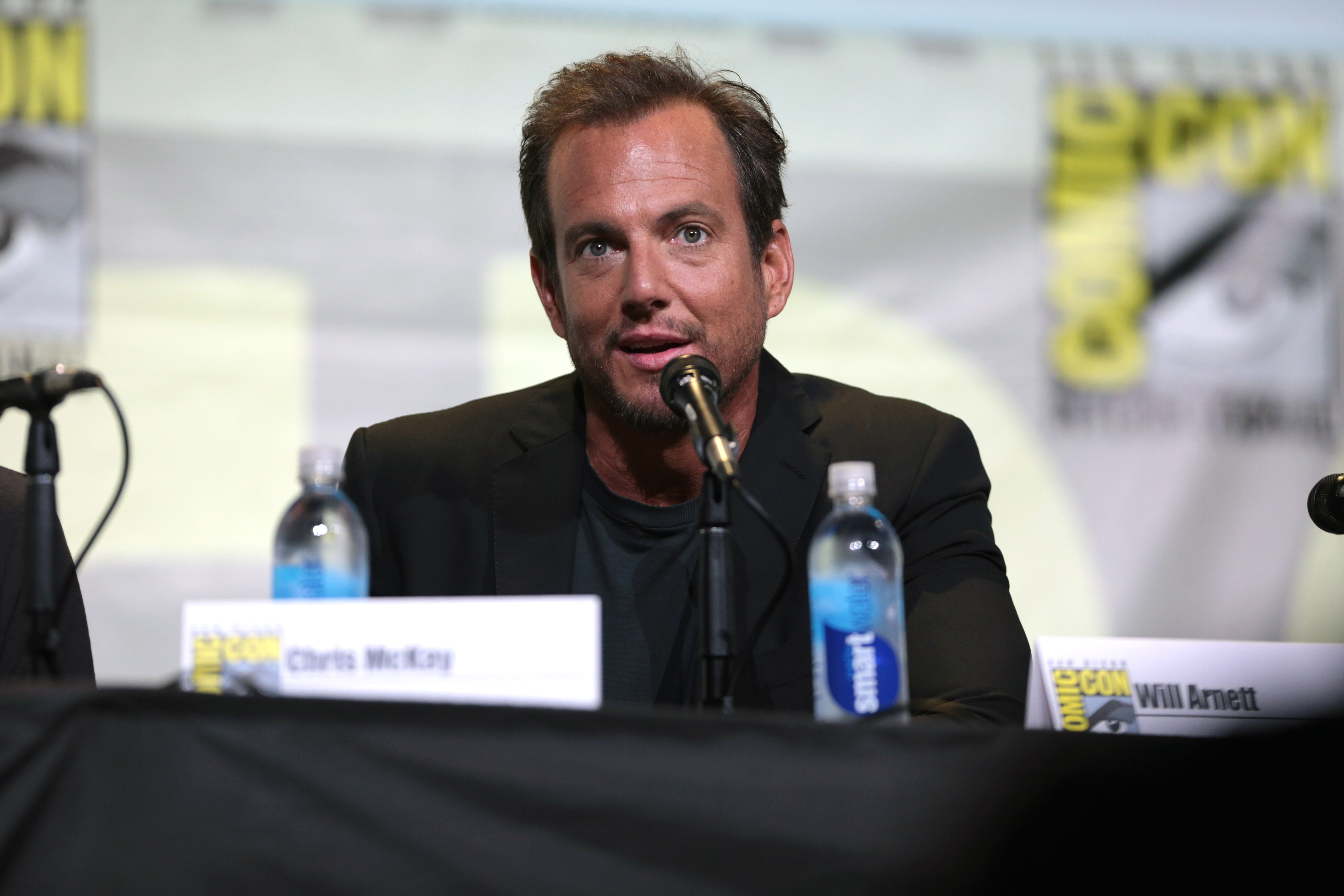In the image, a man with medium-length brown hair, slightly in need of a shave, sits at a table draped in a black cloth. He faces forward, positioned slightly to the left, with light-colored eyes and a suntanned complexion. He wears a dark blazer over a black t-shirt. In front of him, on the table, is a microphone on a small stand, positioned just in front of his mouth.

To the right of the microphone, there is a plastic water bottle and a white card that reads "Comic-Con" with the name "Will Arnett." On the left side of the microphone, another card, slightly out of focus, bears the Comic-Con symbol and the name "Chris McKay." Another water bottle is visible behind this card. The table also has another microphone extending out of the frame on the left side.

The background is a wall adorned with Comic-Con posters, featuring "Comic-Con" in white, gray, and yellow lettering. This setup indicates that the image captures a moment from a Comic-Con event where Will Arnett is featured.